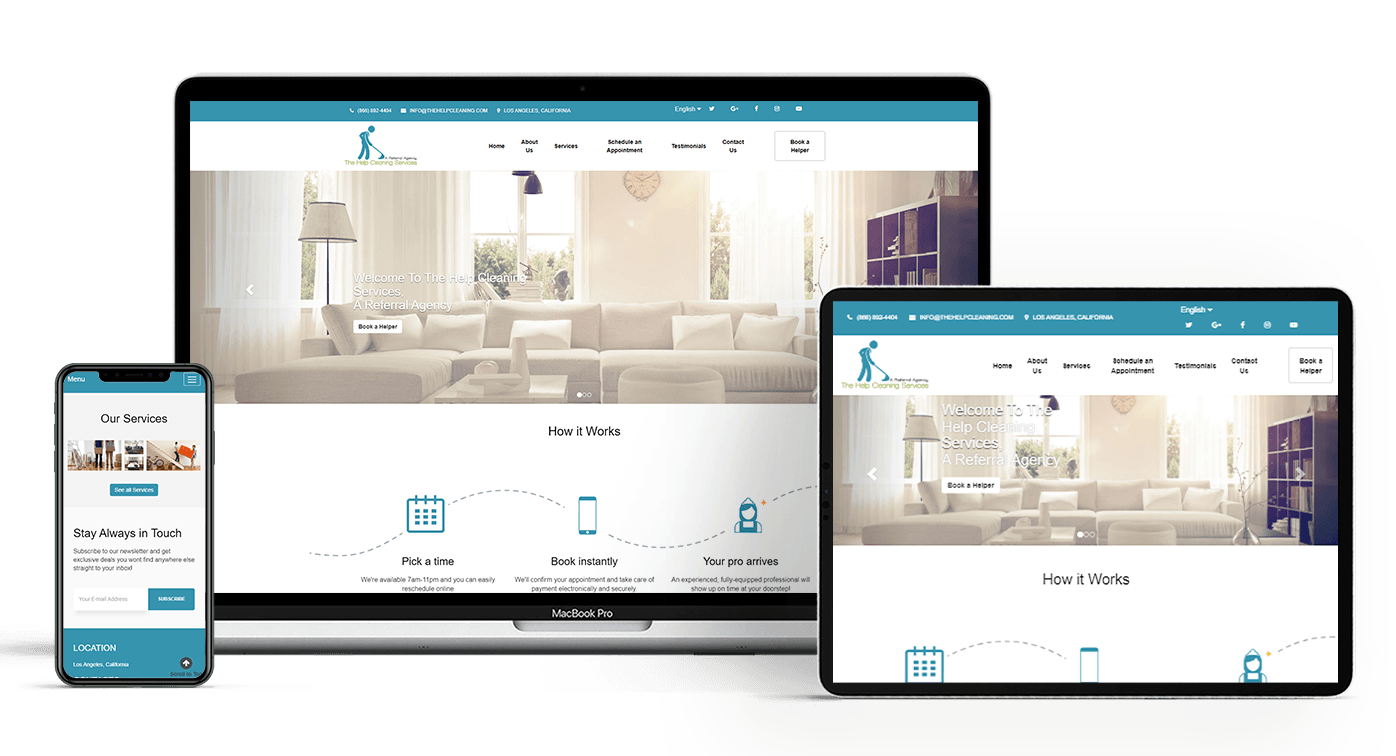This image showcases the responsive design of a website displayed on three different Apple devices: an iPhone on the left, a MacBook Pro in the center, and an iPad on the right. The website maintains a cohesive color scheme and design across all devices, though there are notable differences in layout and content presentation. 

In the center, the MacBook Pro prominently features a clean white and light blue website interface. The focal point of this display is a detailed image of a living room adorned with white couches, white ottomans, white pillows, and white lamps, accompanied by a brown bookcase on the right side. Underneath this scene, a section titled "How It Works" is displayed. 

This section includes illustrations and text describing the process: a calendar icon labeled "Pick a Time" with a note indicating availability from 7 to 11 p.m., followed by a dotted line connecting three steps. The first step emphasizes easy online reachability, followed by a "Book Instantly" prompt featuring a phone icon. The final step, marked by the continuation of the dotted line, leads to "Your Pro Arrives."

To the left, the iPhone screen presents a different layout, characterized by a more blue dominant color palette. Unlike the MacBook Pro and iPad, the living room image is absent. The iPad, on the right, mirrors the MacBook Pro's layout more closely, preserving the same visual and textual elements, reinforcing the consistent design experience across larger screens. 

Overall, this image effectively demonstrates the adaptability and consistency of the website's design across various devices, ensuring a seamless user experience regardless of the platform.